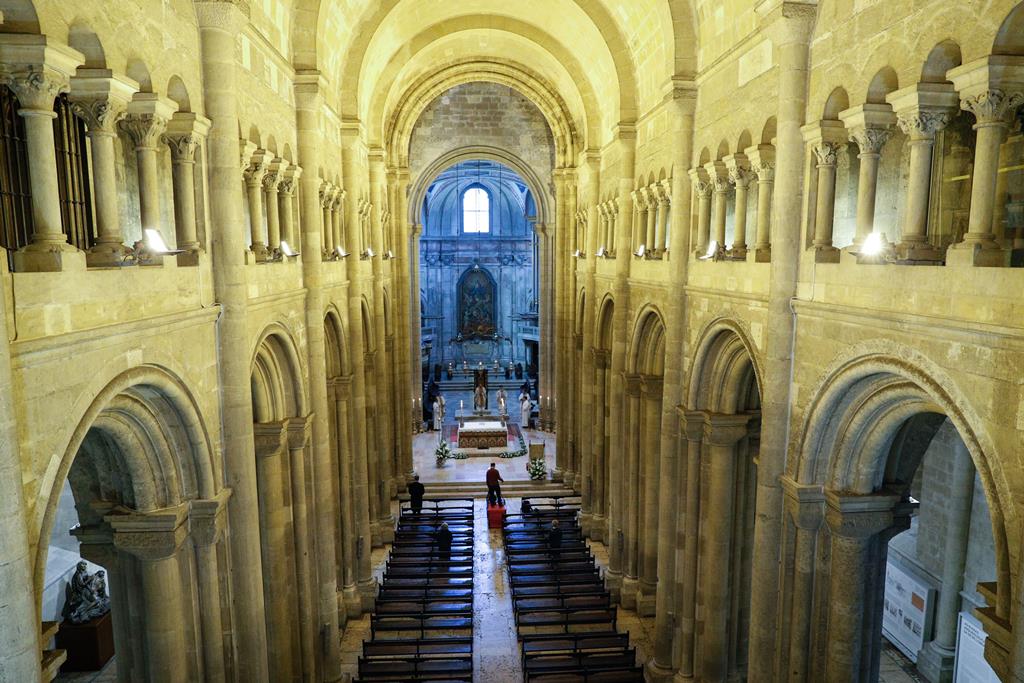The image depicts the grand interior of a cathedral as viewed from a high balcony. The cathedral is characterized by its immense height, with towering stone columns and archways forming two distinct levels—the larger archways at ground level and smaller ones on the balcony. The arched ceilings further accentuate the height and regal essence of the sanctuary. Below, two rows of pews stretch toward an ornate altar area at the front, flanked by a solemn group of at least six individuals clad in white, possibly priests or holy men performing a ceremony. A faint painting or artwork can be discerned behind the altar, and a bright window at the very back streams white sunlight into the expansive stone interior. The space is further adorned with statues, candles, and hanging lamps, with railings and kneeling pads adding to the sacred ambiance. The scene is imbued with a palette of neutral stone tones, dark pews, and the deep blue hues of the distant altar area, creating a solemn yet majestic atmosphere.